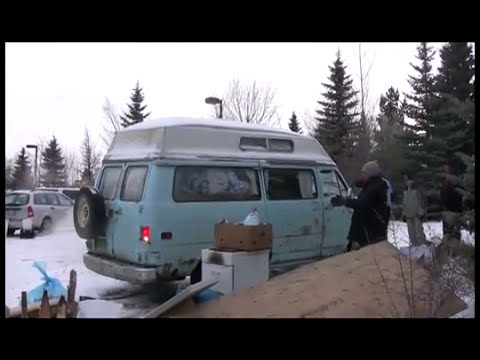The image captures a snowy parking lot scene on a bright yet cloudy winter day. The lot, surrounded by pine trees and illuminated by lampposts, features an old, light blue van with a white roof and a rusty finish. The van, which has a spare tire mounted on its back, appears to have a somewhat elevated roof, possibly suggesting an additional sleeping area. The ground, covered in snow, obscures any markings or spaces typically found in a parking lot. 

Adjacent to the van, on the passenger side, stands a man wearing a tan beanie and a black coat. In front of him, there are a few boxes and what looks like a large piece of wood. Further away, slightly obscured by distance, are two more individuals; one dressed in a black coat and the other in a gray coat. Additionally, scattered throughout the parking lot are other vehicles. To the side of the image, something vaguely human-shaped, possibly a small statue, can be seen. The sky overhead appears completely white, emphasizing the wintry atmosphere.